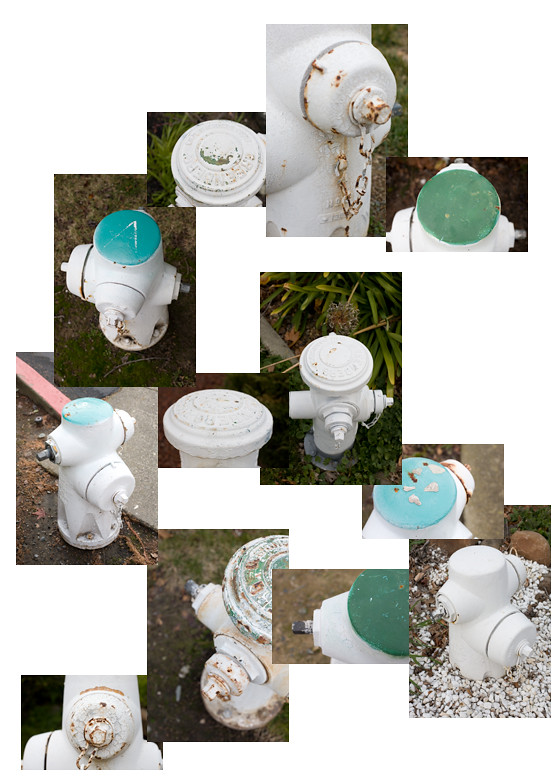The image is a digital collage of color photographs, meticulously arranged in an overlapping S-shape pattern, depicting various fire hydrants. Each photograph showcases a different perspective of white fire hydrants, capturing them from the side, above at a 45-degree angle, or other unique angles. The backgrounds of these photographs vary, featuring grey gravel, brownish soil, green grass, and dark green foliage, with one instance showing a pale yellow line. Most hydrants are worn, exhibiting rust, flaking paint, and other signs of age. A notable detail includes the colorful caps on the hydrants, which are predominantly turquoise, pale blue, or dark green. Despite the digital collage’s overlapping nature, some white background remains visible, enhancing the fragmented yet cohesive display of the hydrants.